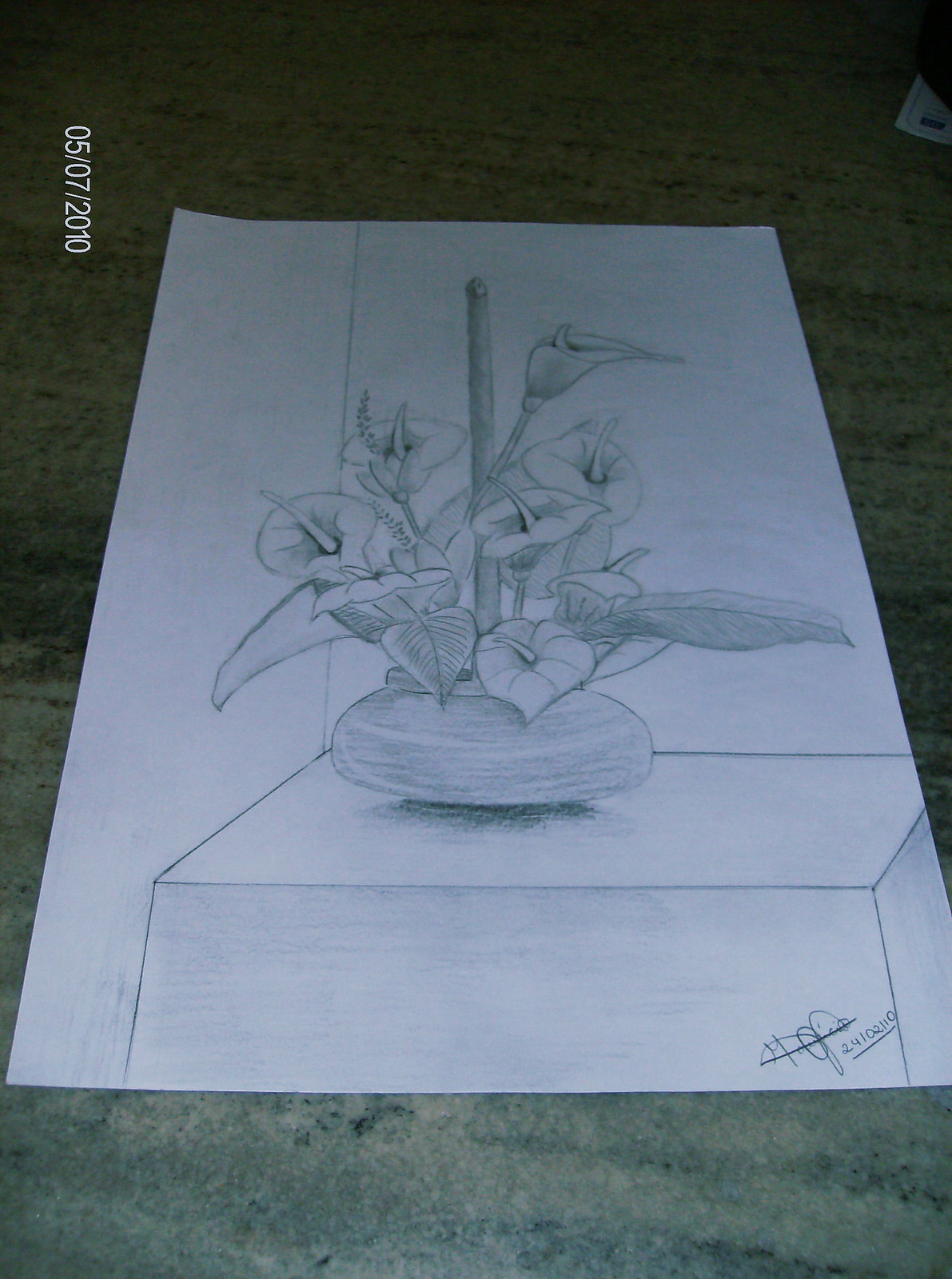This photograph captures a detailed pencil drawing rendered on a pristine white page, resting atop a gray and tan marble or granite surface. The focal point of the drawing is a small square table positioned in the corner of a room, framed by walls on the left and in the background. Atop the table sits a round vase, elegantly housing a cluster of calla lilies. The flowers, distinguished by their slender stems and distinctive cup-shaped, teardrop-like blooms with a single protruding stamen, rise gracefully from the vase. Complementing the blossoms are several oblong, veined leaves nearer to the vase's base, as well as a slightly thicker central stem extending upward, adding depth and balance to the composition.